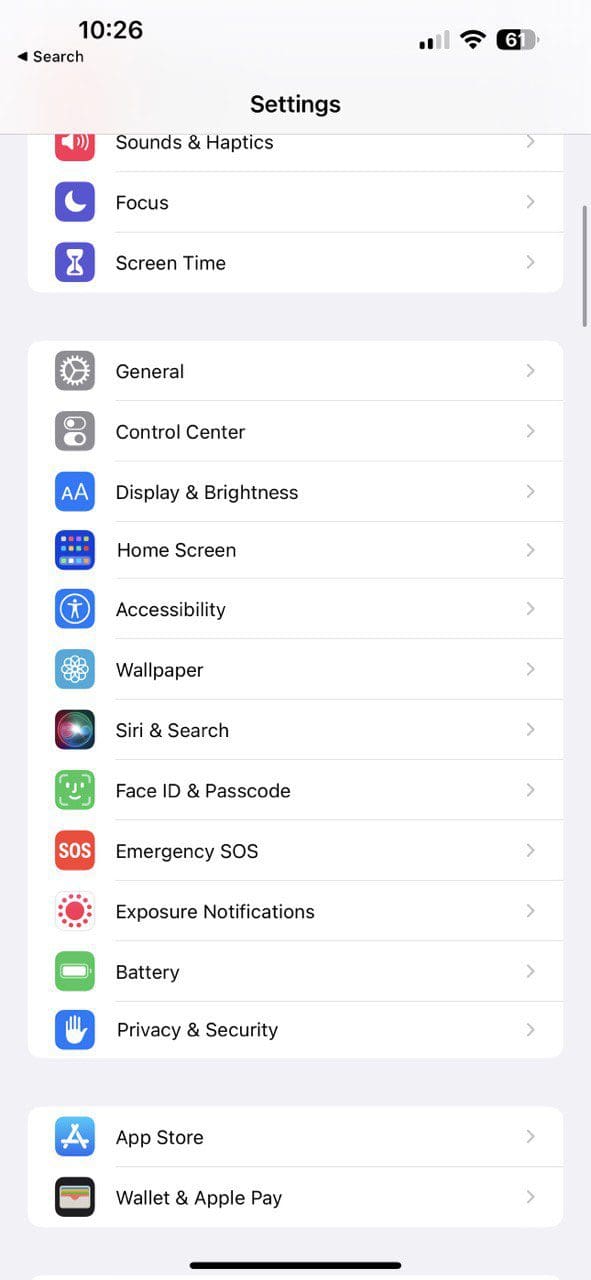This image is a detailed screenshot of an iPhone's Settings menu. The background has a subtle gray outline, emphasizing the semi-transparent gray menu situated at the top of the screen. In the upper left corner, the time reads "10:26" in black text. Directly below that, there is a "Search" option accompanied by an arrow pointing to the left, indicating a back navigation option. Centrally positioned at the top of the screenshot is the word "Settings" with a capital "S". On the upper right, several status indicators are displayed: the mobile phone signal shows two out of four bars, the Wi-Fi signal indicates full connectivity with three bars, and the battery icon reveals a charge level of 61%.

Beneath these status indicators, the main section of the Settings menu displays a series of options in white rectangular boxes, each with an accompanying icon, black text, and a gray arrow pointing to the right. The visible options include "Sounds & Haptics", "Focus", and "Screen Time". As the user scrolls further, additional options present themselves: "General", "Control Center", "Display & Brightness", "Home Screen", "Accessibility", "Wallpaper", "Siri & Search", "Face ID & Passcode", "Emergency SOS", "Exposure Notifications", "Battery", and "Privacy & Security".

Following a slight gap that reveals more of the gray background, the final listed options are "App Store" and "Wallet & Apple Pay". At the very bottom of the screen, a small black line is centered, likely indicating the bottom boundary of the menu display. This comprehensive view encapsulates the typical layout and structure of the iPhone's Settings menu.